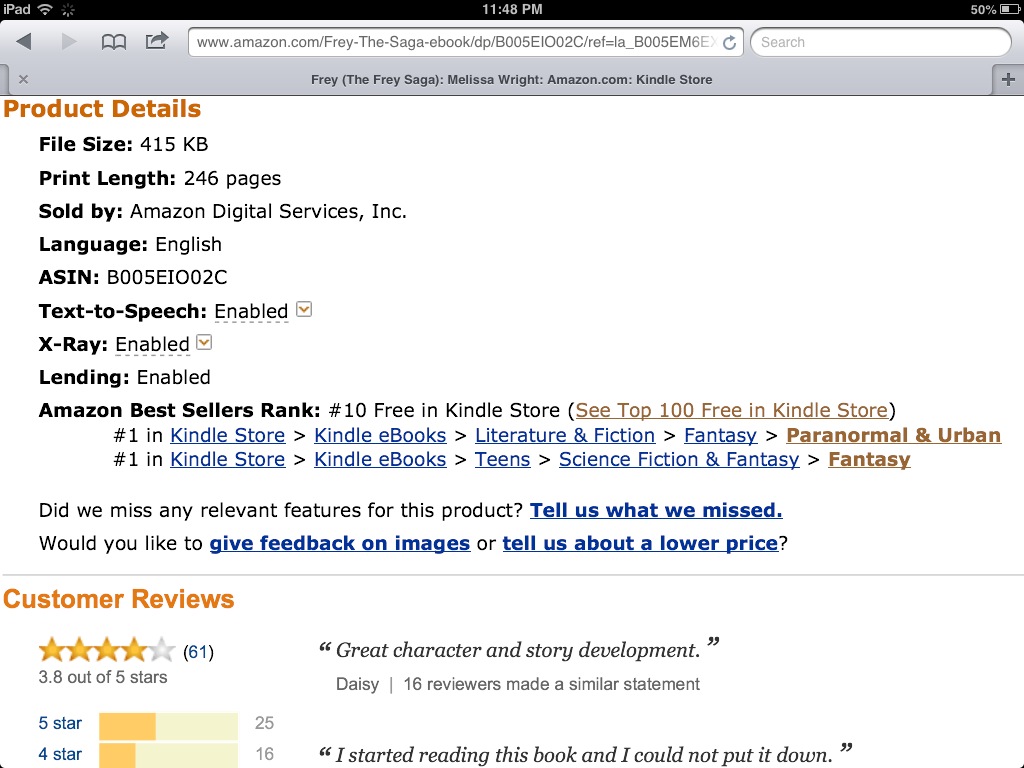**Detailed Image Description:**

The image showcases a webpage displayed on an iPad screen. At the top of the screen, there is an iPad header bar indicating a Wi-Fi connection, the time as 11:48 PM, and the battery level at 50%. 

The webpage appears to be an Amazon product page for an ebook titled "Fray: The Saga." Various details about the ebook are listed, including:

- **File Size:** 415 KB
- **Print Length:** 246 pages
- **Sold By:** Amazon Digital Services Inc.
- **Language:** English
- **ASIN:** B005EIO02C
- **Features:**
  - Text-to-Speech: Enabled
  - X-Ray: Enabled
  - Lending: Enabled

The ebook ranks as follows in Amazon's Kindle store:

- **Amazon Best Sellers Rank:** 
  - #10 in Free in Kindle Store
  - #1 in Kindle Store > Kindle eBooks > Literature & Fiction > Fantasy > Paranormal & Urban
  - #1 in Kindle Store > Kindle eBooks > Teens > Science Fiction & Fantasy > Fantasy

Below the product details, there's a prompt asking if any relevant product features were missed, inviting users to give feedback, submit images, or report a lower price.

Further down, the **Customer Reviews** section is displayed prominently in orange, showing:

- **Overall Rating:** 3.8 out of 5 stars
- **Detailed Breakdown:** 
  - 4 out of 5 stars emphasized in yellow, based on 61 reviews.
  - 25 users gave 5-star reviews.
  - 16 users gave 4-star reviews.
- Highlighted Customer Comments:
  - "Great character and story development." - Daisy (agreed upon by 16 reviewers)
  - "I started reading this book and I could not put it down."

The majority of the webpage features a clean design with a white background, black text, and key elements highlighted in orange.